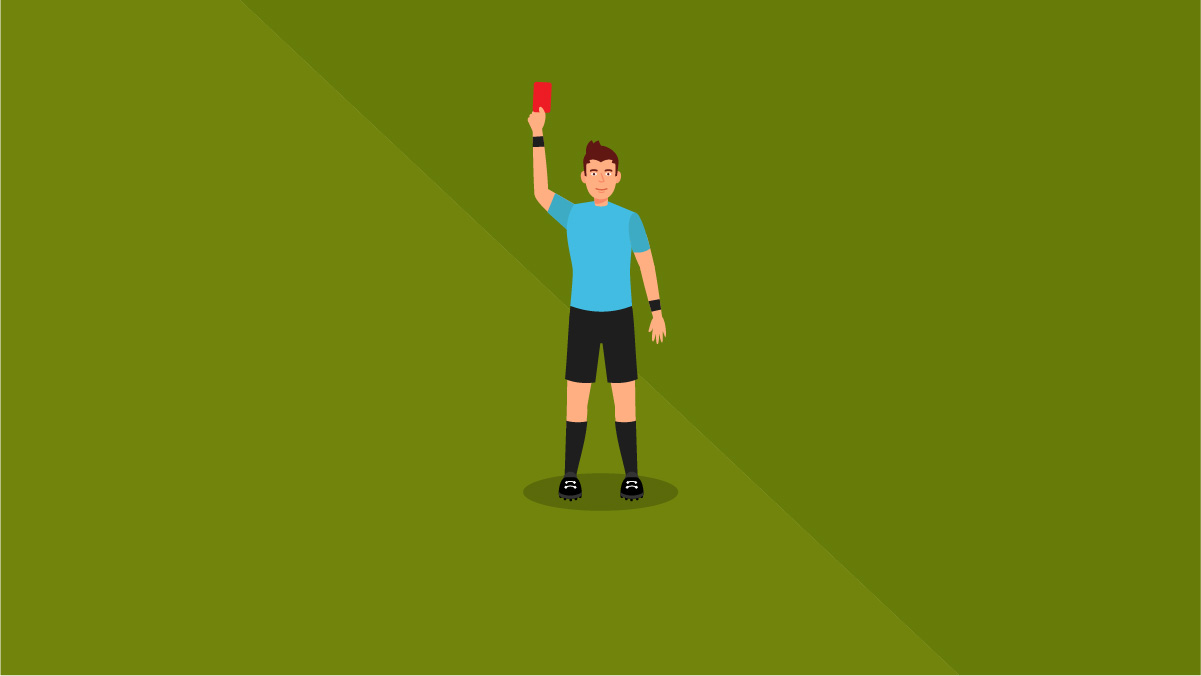The image features a computer-generated depiction of a football referee standing against a green background that is diagonally divided into a darker upper right portion and a lighter lower left portion, resembling a soccer pitch. The referee, appearing as an icon-like avatar, is centered within the composition and casts a circular shadow, suggesting it is a sunny day. He is dressed in a blue jersey, black shorts, black socks, and black cleats with white shoelaces. Both of his wrists sport black wristbands, and he wears a watch on his left wrist. The referee has short brown hair and is holding a red card high in his right hand.